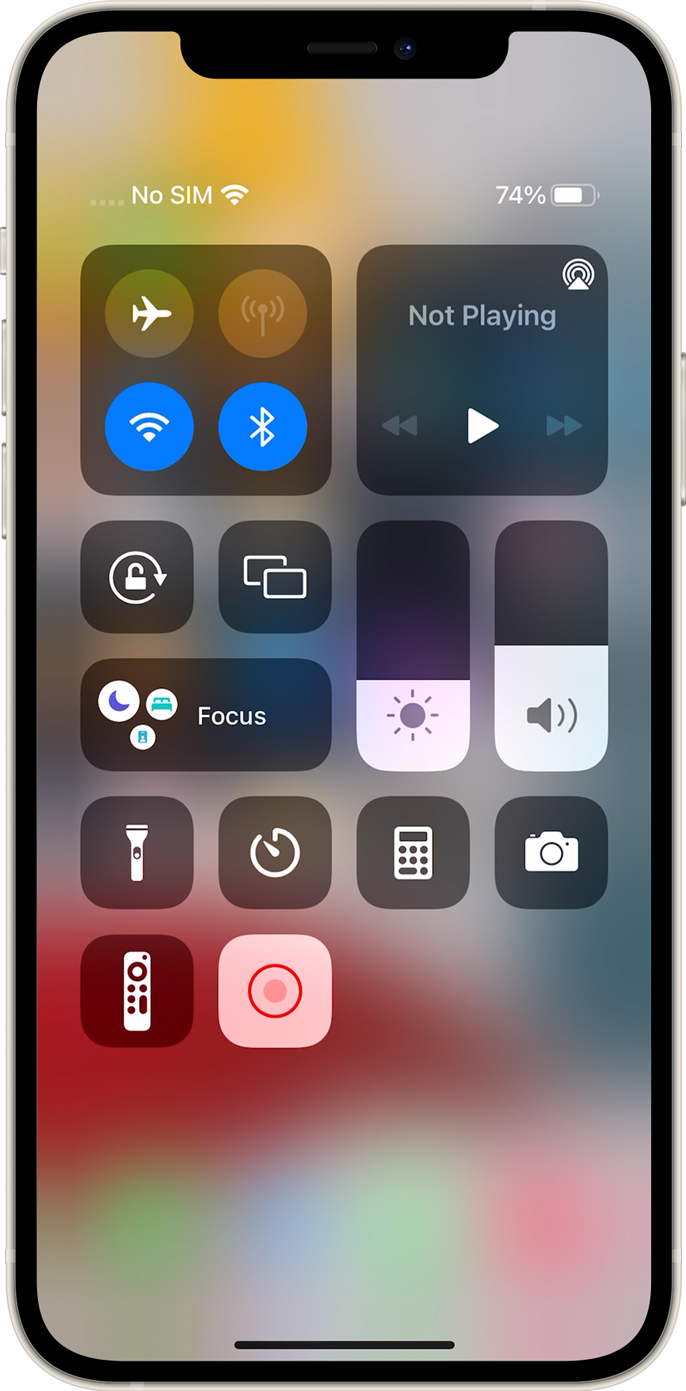This detailed caption describes the user interface of an iPhone as seen in an image:

The image showcases the front interface of an iPhone. The phone is encased in a sleek black border with a barely visible power button and volume controls on the left side, and another button, typically used for turning the screen off, on the right side. At the top, the black border subtly slopes down to accommodate the front-facing cameras. At the bottom, there's a black bar that can be swiped up to access more features.

On the screen, in the top left corner, white text displays "No SIM" alongside a full Wi-Fi signal strength indicator. Near the top-right corner, the battery icon shows 74% charge in white.

The main control center of the iPhone consists of several organized sections. The first box has four icons arranged in a 2x2 grid. The top row includes icons for Airplane Mode and Personal Hotspot. The bottom row features icons for Wi-Fi and Bluetooth, both of which are currently enabled.

To the right of this box, there is a media player widget labeled "Not Playing," containing controls with previous track, play/pause, and next track buttons.

Below the first box, the screen displays the text "Unlock." Following this, there is a second box showcasing multiple screen thumbnails.

Below, a bar dedicated to "Focus" settings spans across the screen, containing three icons. To the right of this bar are two vertical sliders: one for screen brightness, which is set to a very low level, and one for volume, set to about halfway.

Four additional utility icons stretch across below these sliders: Flashlight, Timer, Calculator, and Camera. Below these, two more icons are observed: a remote control icon and a red circle with a lighter red center, likely indicating a recording feature. 

The background of the screen is an aesthetically blurred swirl of numerous colors, adding a vibrant and dynamic feel to the interface.